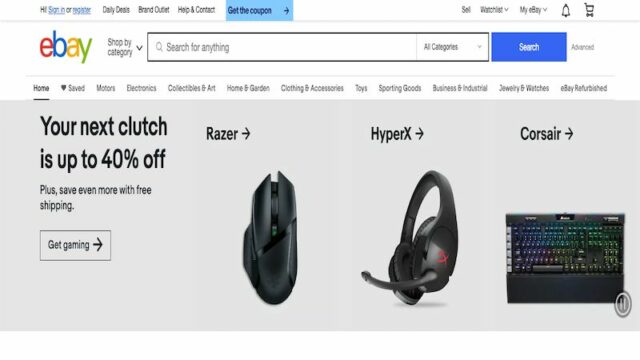This image appears to be a detailed screenshot of the eBay website, showcasing various navigation options and promotional content. At the top, there is a distinctive white header featuring the eBay logo, alongside options like "Sign In," "Deals," "Brand Outlets" (possibly misspoken as "brand outfits"), "Help & Contact," and a prominent blue button labeled "Get the Coupon." Adjacent to these options, there are links for "Sell," "Watchlist," "My eBay," notifications, and a shopping cart icon.

Just below the main header, the eBay logo is displayed again, followed by a comprehensive search bar with a category filter and a blue search button, accompanied by an "Advanced" search option. Beneath this search functionality, another navigation bar is present, listing categories such as "Home," "Saved," "Motors," "Electronics," "Collectibles & Art," "Home & Garden," "Clothing & Accessories," "Toys," "Sporting Goods," "Business & Industrial," "Jewelry & Watches," and "eBay Refurbished."

The bottom portion of the image has a gray background with promotional text stating, "Your next clutch is up to 40% off, plus save even more with free shipping. Get gaming." Here, popular brands like Razer, HyperX, and Corsair are highlighted. Below the brand names, images of specific gaming accessories are displayed: a black Razer mouse, a black and red HyperX headset, and a black Corsair keyboard featuring a rainbow backlight. This detailed layout encapsulates not only the website's structure but also its current promotional focus.